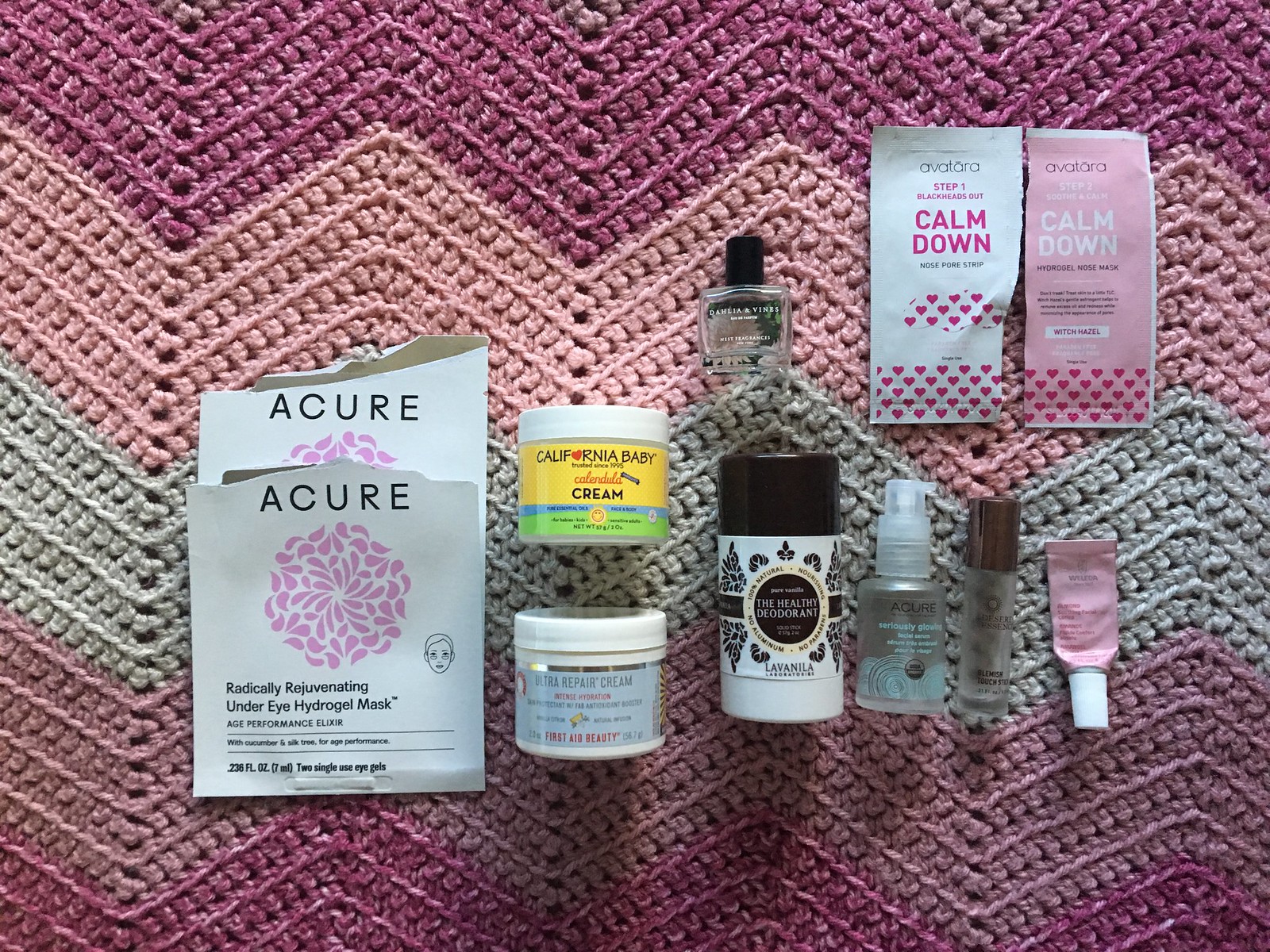In the background of the image, there is a soft, gradient fabric showcasing hues of purple, pink, and light blue, creating a serene and calming atmosphere. On a coffee table in the foreground, several items are meticulously placed. To the left, there is an open "Under Eye Hydrogel Mask" labeled "Cure Rejuvenation," decorated with small, delicate white flower petals. The mask's packaging features a minimalist design with a silhouette of a face. 

To the right of this mask, there are two more packets - the left one is white adorned with tiny hearts, while the right one is pink with similar heart motifs. Surrounding these packets are several small, clear bottles that are difficult to read due to their light blue and dark text.

Additionally, there is a well-used pink tube, indicative of its frequent usage. Adjacent to it stands a white canister with a black pop-top, labeled "California Baby Cream," featuring a white lid and a light blue label. Another container with a white lid and additional text is slightly visible, adding to the assortment of skincare and beauty products displayed on the table.